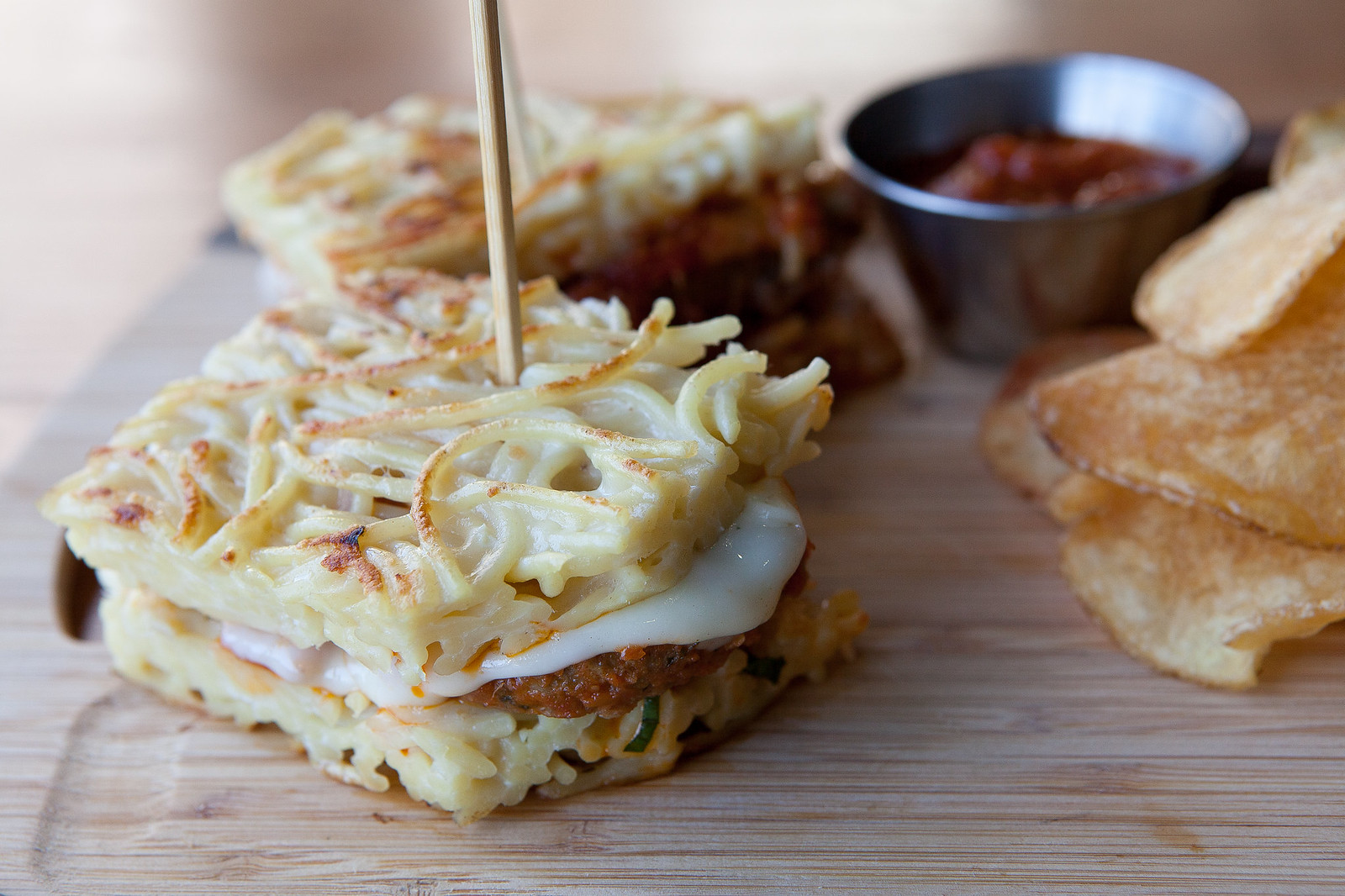The photograph features a light-colored, almost white wooden cutting board with distinct horizontal wood grain patterns. In the upper right corner of the cutting board, there's a small, silver bowl containing a vibrant red sauce. Just below the bowl, a handful of homemade potato chips are spread out. These chips are thinly sliced, with their dark-colored peels still intact along the edges, giving them a rustic, homemade appearance. The chips are browned and look delectably crispy.

At the top left of the cutting board, there is an out-of-focus sandwich, but as the eye moves downward, the camera's focus reveals more details. The sandwich features buns made of crispy browned spaghetti noodles congealed with white cheese. Nestled between these unique buns is a piece of browned meat with melted white cheese oozing down its side. Near the top of the sandwich, a wooden toothpick is lodged, holding the structure in place.